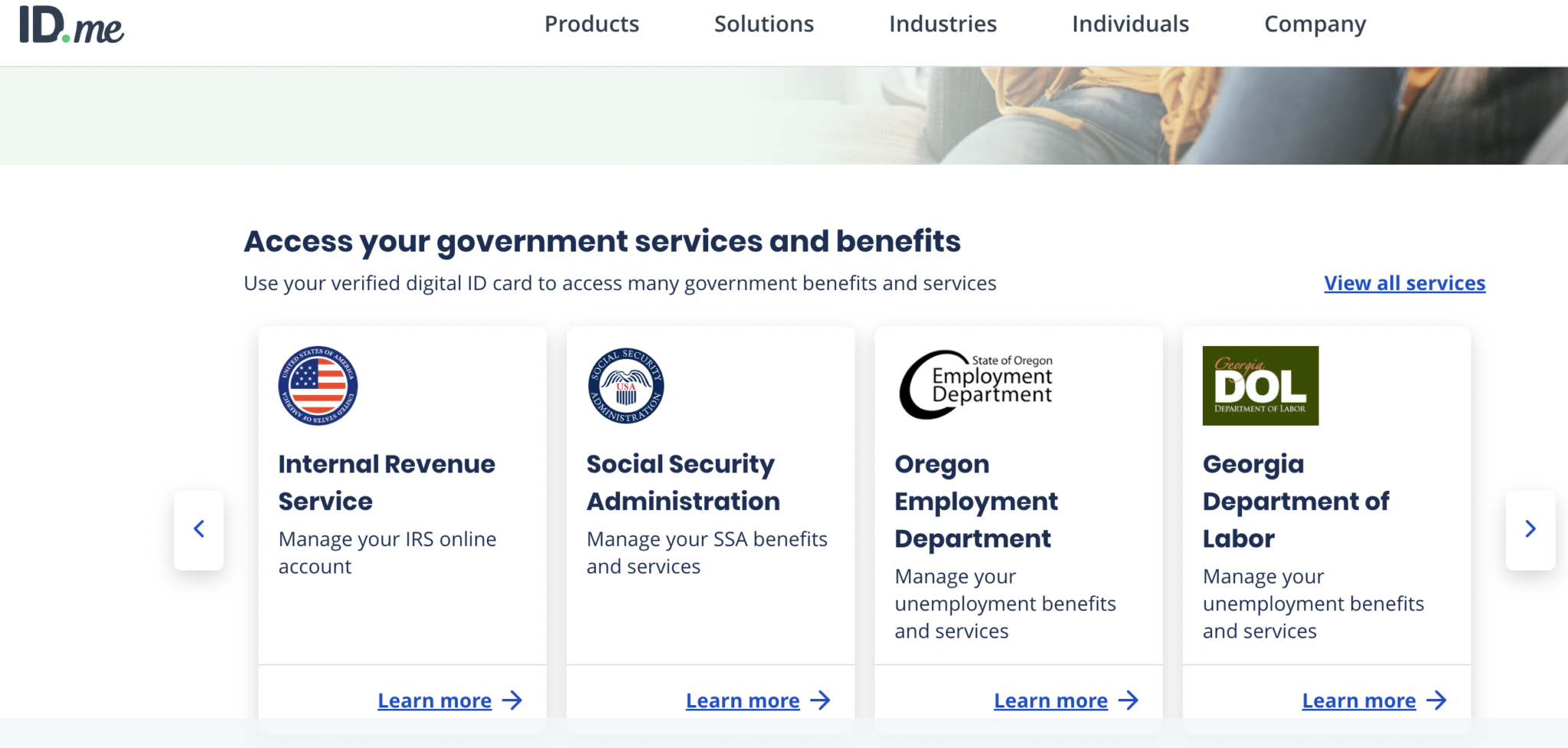This image is a screen capture from a computer interface. In the top left corner, the logo "ID.me" is displayed with a green dot beside it, indicating an active status. Spanning across the top of the screen, starting slightly before the halfway mark, are navigation categories labeled as "Products," "Solutions," "Industries," "Individuals," and "Company."

The upper portion of the screen contains a narrow strip of an image, primarily shaded in a light mint green hue. The image appears to show someone sitting on a couch, with their legs faintly visible. Below this image, a prominent message reads, "Access your government services and benefits. Use your verified digital ID card to access many government benefits and services." To the right of this message, a hyperlink labeled "View all services" is prominently displayed.

On either side of the screen, navigation buttons are visible: a back arrow on the left and a forward arrow on the right. Below this section, four categories are listed, each with a brief description and a "Learn more" hyperlink in blue:

1. **Internal Revenue Service**: Manage your IRS online account.
2. **Social Security Administration**: Manage your SSA benefits and services.
3. **Oregon Employment Department**: Manage your unemployment benefits and services.
4. **Georgia Department of Labor**: Manage your unemployment benefits and services.